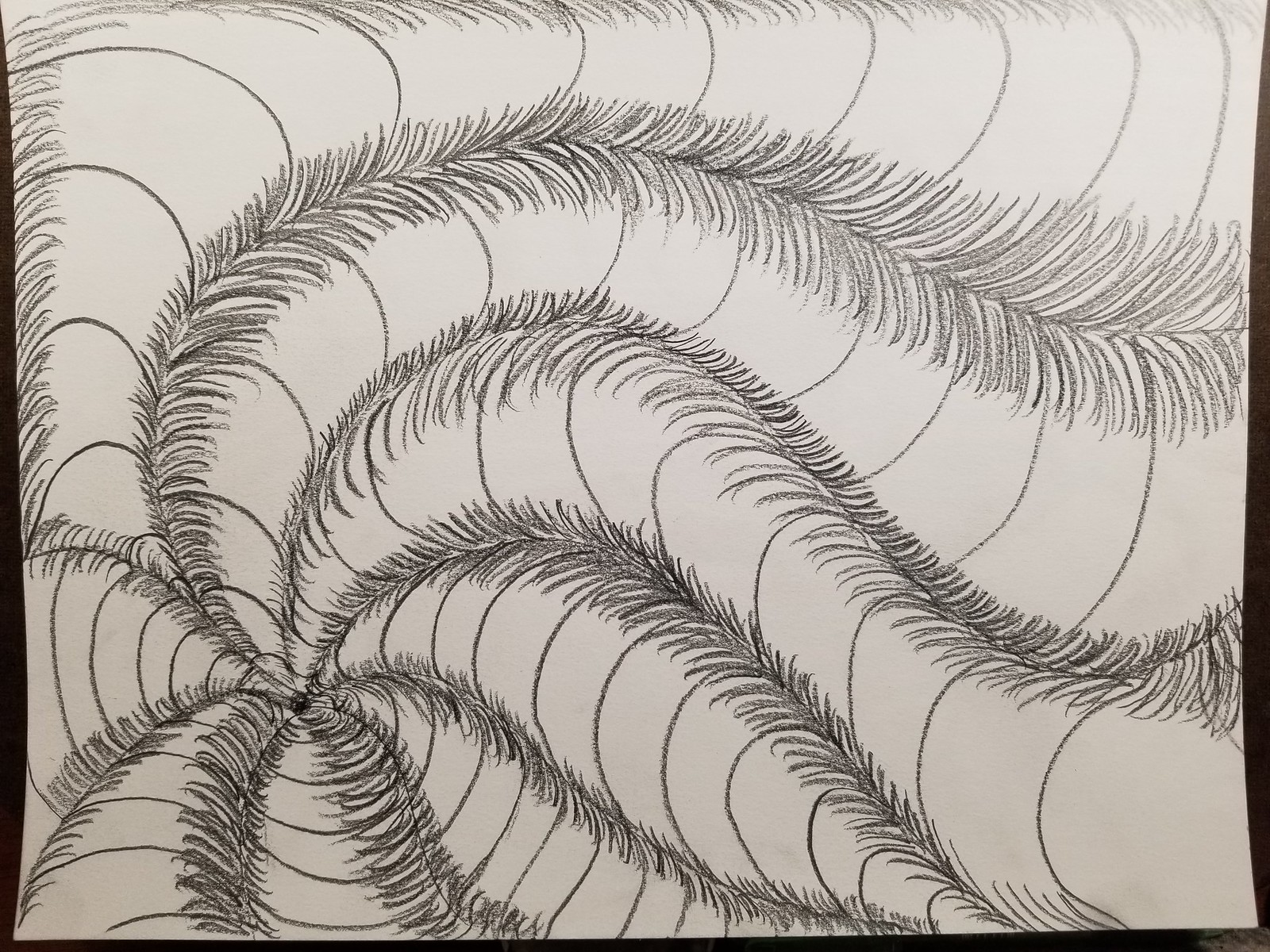This photograph showcases a detailed black and white sketch on a white piece of drawing paper. The drawing originates from a small black dot located towards the lower left side of the paper, just about an inch away from the edge. From this dot, there are eight cylindrical, curved lines radiating outward in various directions, creating an intricate and swirling pattern. These intricate lines, resembling the tentacles of an octopus or perhaps feathery leaves, exhibit a mesmerizing play of thin and thick black marks. The lines protrude from the central dot, spreading to the left corner, top right, top left, and bottom right, with one particularly elaborate line winding completely around from the center left to the top right. Surrounding the pattern, the paper features a black strip along the left, right, and bottom edges, which frames the drawing, adding a sense of depth and contrast. The artist's technique, possibly using a black colored pencil, has created a rich texture, with some segments showing densely packed feathery or hairy details, giving the entire sketch a complex and organic feel.